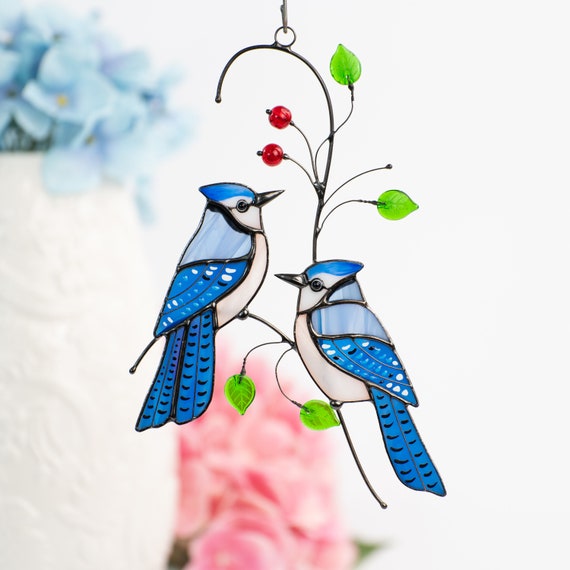This image features a close-up photo of a decorative hanging ornament. The central motif is a delicately crafted metal branch adorned with beads, designed to resemble a natural scene. The branch, with its spiraling metal and numerous offshoots, supports four bright green stained glass leaves and two small red berries made from beads. Perched on the lower section of the branch are two beautifully detailed stained glass blue jays. These birds exhibit varying shades of blue, with dark blue adorning their head and tail feathers, and a light sky blue coloring their mid-back. One blue jay seems to be gazing upward at a red berry, while the other bird appears to be looking affectionately at its mate. The background of the image is intentionally blurred, predominantly white, but hints of blue and pink flowers are visible, adding a subtle yet charming depth to the scene.